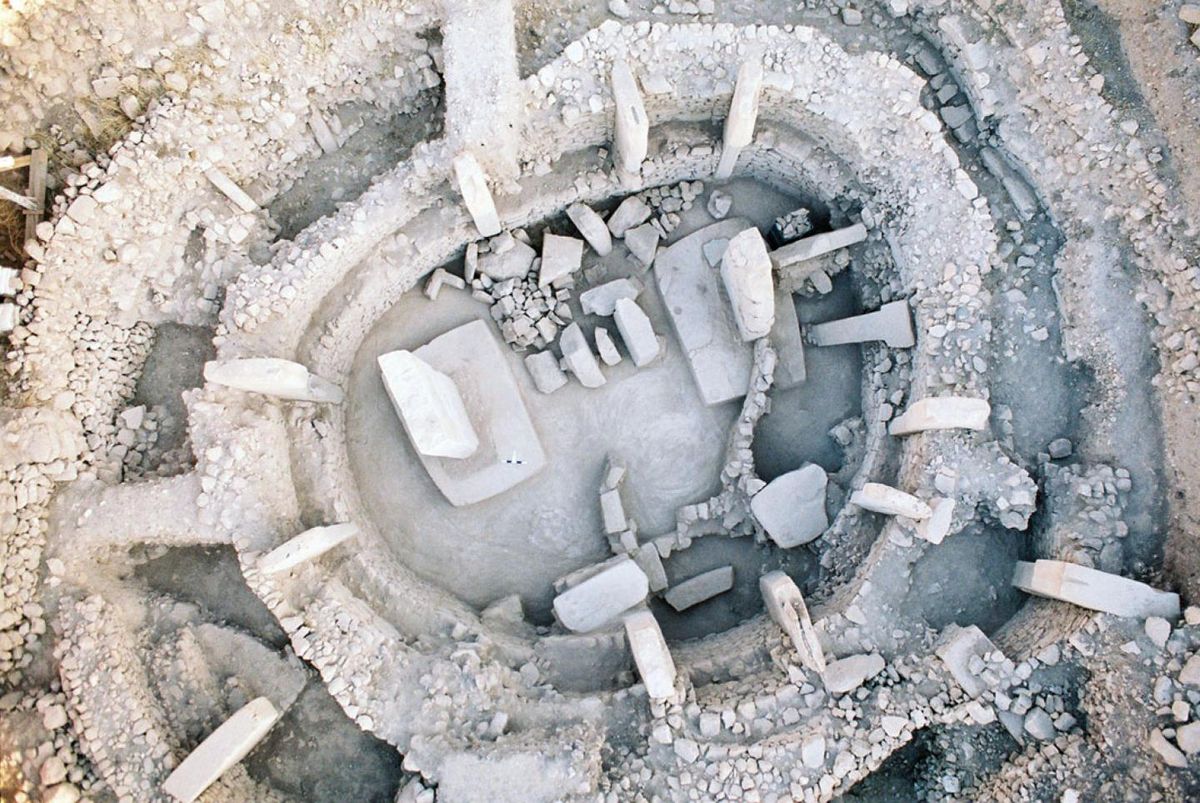This aerial photograph captures an ancient archaeological site showcasing a series of concentric stone walls constructed from medium-sized stones forming circular enclosures. The central circular area stands out as notably clean and well-maintained, with tall structural stone slabs that resemble gravestones or large tablets, meticulously arranged in the middle and along the edges. The configuration includes interconnected stone hubs that visually depict a chamber or room laden with polished stone or marble elements, set against a backdrop of varied rock, dirt, and sediment layers. Towards the top left corner, a wooden board, possibly part of the ongoing archaeological project, can be seen, although no other equipment, scaffolding, or personnel are present in the image. The overall color palette consists of muted grays, whites, and ivories, emphasizing the historical and preserved nature of this dig site.